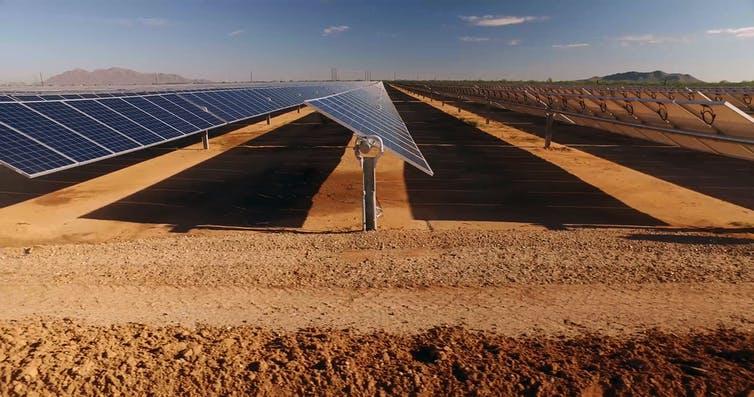The photograph depicts a vast solar farm, appearing professional and poised against a rugged desert backdrop. In the foreground, long rows of solar panels stretch out, their sleek surfaces gleaming blue and tilted at a strategic angle, likely around 45 degrees, to maximize sun exposure. The shadow of each row of panels stops just before the next, and a dirt path runs in front of them. The soil is loose and dusty, suggestive of the arid desert environment. To the left and right, there are occasional hills, and towering in the background is a large, long bridge partially obscured from view, giving a sense of scale and distance. The sky above is a vivid blue, dotted with a few sparse clouds, and further back, mountains rise majestically, with a hint of green foliage at their base, possibly indicating a vineyard. The scene, rich in detail, conveys a sense of futuristic efficiency and natural grandeur, reminiscent of images seen in National Geographic or other environmental magazines.